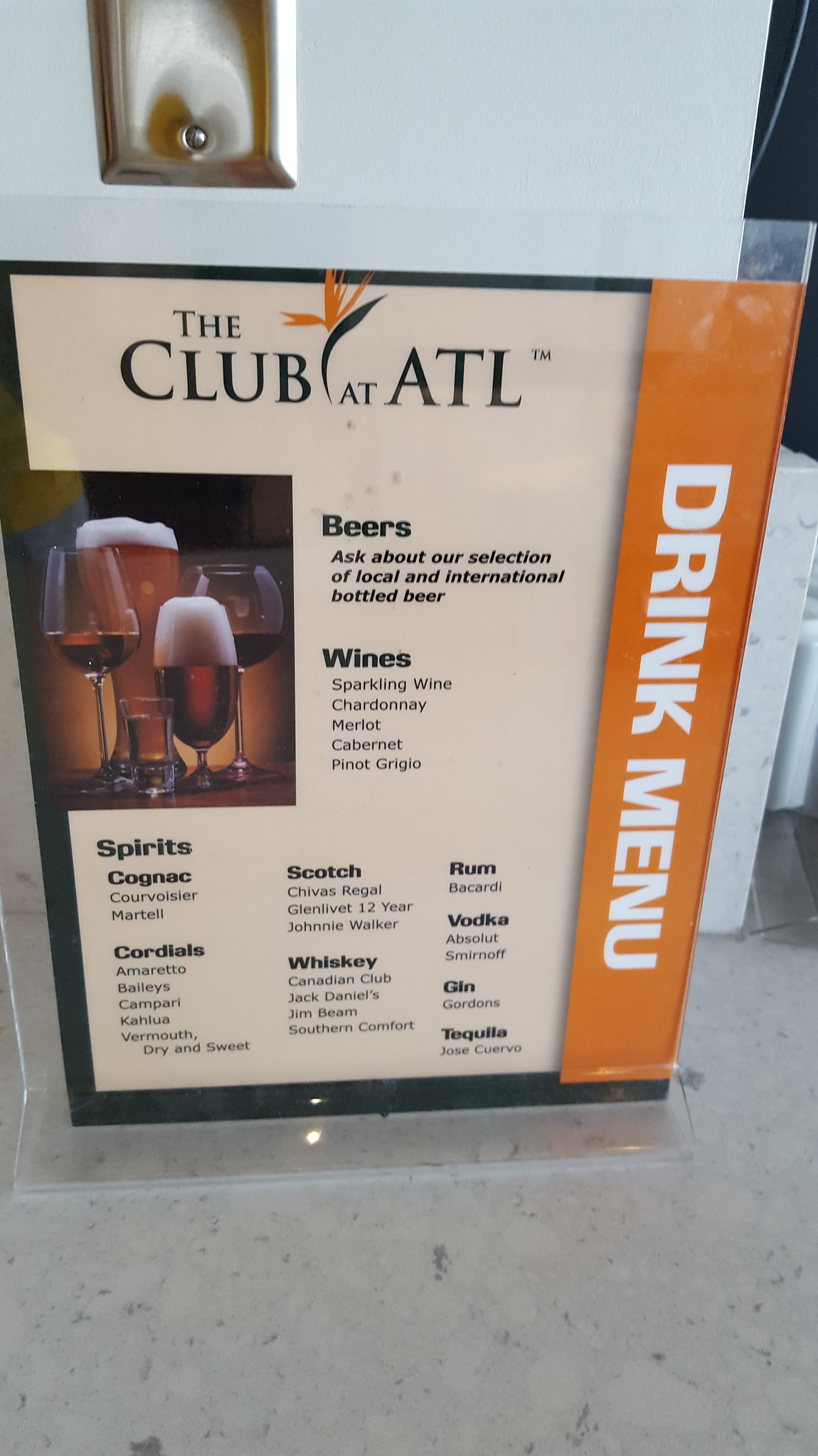The image showcases a freestanding menu display, typical of those found in restaurants or lounges, encased in clear plastic for protection. It stands sturdily against a pale whitish-blue wall, adjacent to an indeterminate silver panel. The primary focus is the menu from "The Club at ATL," presumably located in Atlanta, which details a wide array of alcoholic beverages.

The top left corner of the menu features illustrations of various drink glasses, including beer glasses, wine glasses, and other stemware, indicative of the types of beverages offered. The beverages are listed in three organized columns.

For beers, the menu invites patrons to inquire about their selection of local and international bottled options. The wine section features an assortment of types such as sparkling wine, Chardonnay, Merlot, Cabernet, and Pinot Grigio.

The spirits selection lists several high-end options:
- Cognac: Courvoisier, Martell
- Scotch: Chivas Regal, Glenlivet 12 Year, Johnnie Walker
- Rum: Bacardi
- Vodka: Absolut, Smirnoff
- Gin: Gordon's
- Tequila: Jose Cuervo
- Whiskey: Canadian Club, Jack Daniel's, Jim Beam, Southern Comfort

Additionally, for cordials, the menu includes:
- Amaretto
- Baileys
- Campari
- Kahlua
- Vermouth (Dry and Sweet)

This meticulous drink menu offers a comprehensive look at the beverages provided at The Club at ATL, catering to a variety of tastes and preferences.